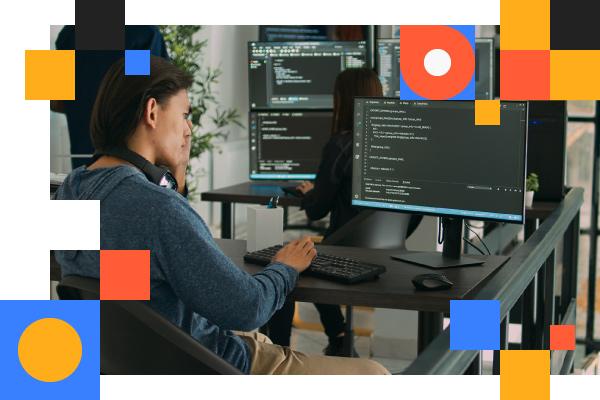This photograph captures an open office space featuring two individuals focused on their work at minimalist desks made of dark wood. The worker closest to the camera is clad in a blue sweatshirt and tan khakis, accessorized with headphones around their neck while engrossed in what appears to be lines of code on a large monitor. Behind them sits another worker, a woman also working on coding, utilizing a stacked dual-monitor setup. The composition is adorned with a variety of geometric forms—squares and circles—superimposed over the image, particularly at the corners. These shapes come in various colors, including red, orange, black, blue, mustard yellow, and rose. Notably, one square features a circular icon with an additional inner circle, enhancing the artistic, design-oriented feel of the photograph.